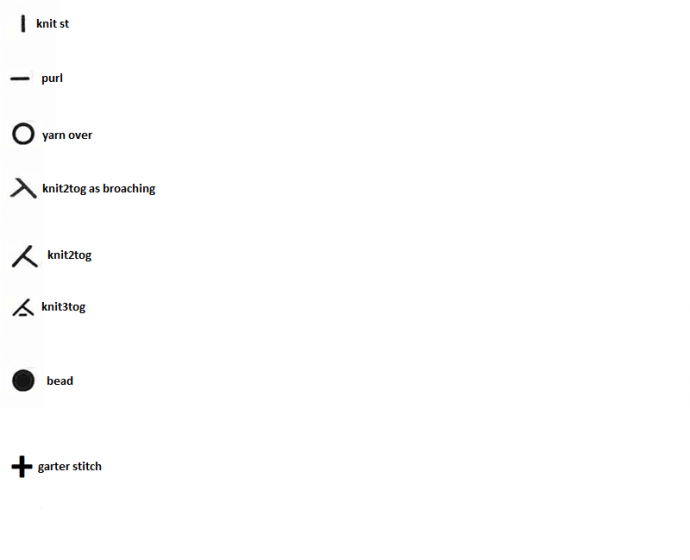The image presents a minimalistic design, set against a pristine white background. On the left side, an organized column of icons or symbols is visible:

1. At the top left, there is a simple vertical black line resembling the number "1." To the right of this symbol, the text reads "Knit Stitch."
2. Directly below, a horizontal line reminiscent of an underscore is depicted. To its right, it is labeled "Purl."
3. Following this, a small round circle appears, with the adjacent label "Yarn Over."
4. Beneath that, the letter "T" leaning to the right is shown. Next to it, the text "Knit Two Together" is indicated.
5. Further down, another "T" leaning to the left is present, accompanied by the caption "Knit Two Through the Back Loop."
6. Below, a "T" that is leaning to the left and paired with an underscore is illustrated, with the label "Knit Three Together."
7. Next in the sequence is a solid black circle, denoted as "Bead" on the right.
8. Finally, a plus sign appears at the bottom with the corresponding text "Garter Stitch."

This clear and concise diagram effectively communicates various knitting symbols and their associated instructions.